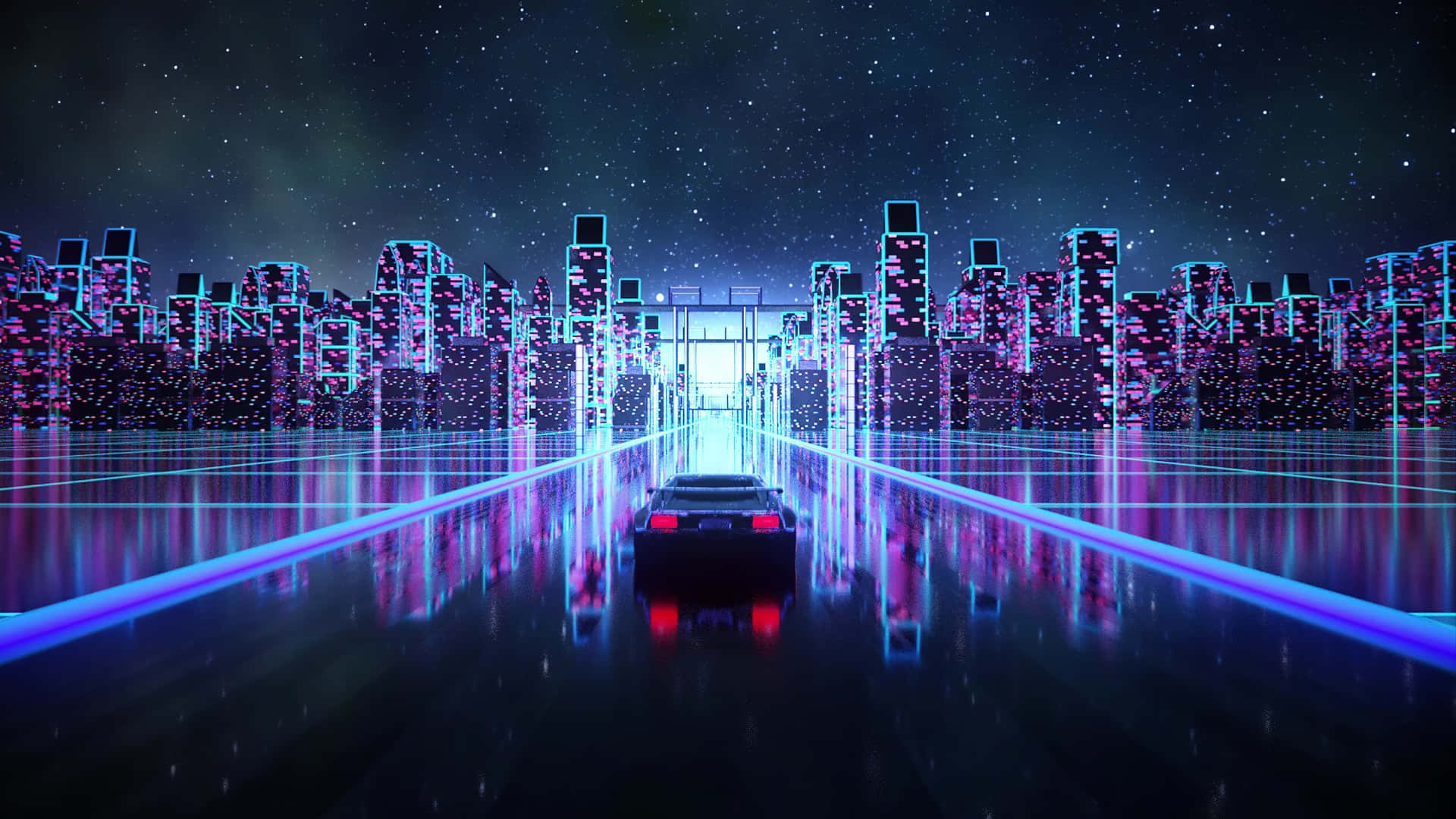This image depicts a highly stylized, futuristic cityscape under a star-studded night sky, filled with shades of green, blue, and black. The foreground features a sleek, black, futuristic sports car with red taillights, positioned on a shiny road that stretches into the distance. Flanking the road are grids illuminated in neon blue. The car appears to be heading toward a city composed of towering, imaginative skyscrapers brightly outlined in neon pink, blue, and purple hues. The surreal cityscape, which appears more like a fantasy rendering or AI-generated image, is adorned with numerous stars, adding to the otherworldly ambiance of the scene.